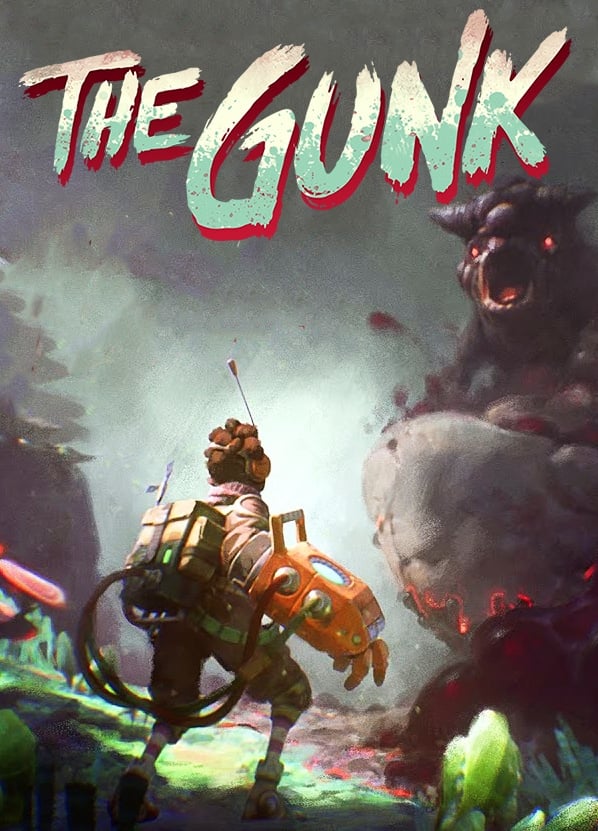This image is a striking piece of concept art, likely a cover for a comic book or a science fiction graphic novel. The art style is reminiscent of a cartoon-like graphic novel with a vertical rectangular frame. The background features a cloudy, smoky gray sky that transitions into a white glow toward the middle and bottom of the image, amplifying its dramatic effect.

Dominating the upper part of the image, in painted, faded letters, are the words “THE GUNK.” The text blends hues of red, white, and a light teal, with a distinctive red drop shadow that emphasizes its prominence. The letters appear as if they were written with a paintbrush or a paint marker, adding to the hand-crafted feel of the poster.

In the foreground, a smaller human-like character stands with an assertive posture, facing a massive creature on the right. This character is equipped with a conspicuous mechanical orange arm that has hoses in red and green connected to a corresponding backpack. The backpack, intricate in design, features a hose and possibly other mechanical appendages. The character also wears orange and white headphones with an antenna, further accentuating their futuristic appearance.

In stark contrast to the small character, a large, stone-like monster looms on the right side. This colossal creature has glowing red eyes and a large, menacing open mouth with something glowing within. The lower part of the monster seems to resemble molten lava, adding to its fiery, volcanic demeanor. The scene is further enriched with green crystals and rocks on the ground, each detail contributing to the fantastical environment.

The overall imagery evokes a classic David and Goliath scenario, where the illuminated, vibrant smaller character stands bravely against the daunting, dark monster amidst a smoky, ethereal backdrop.